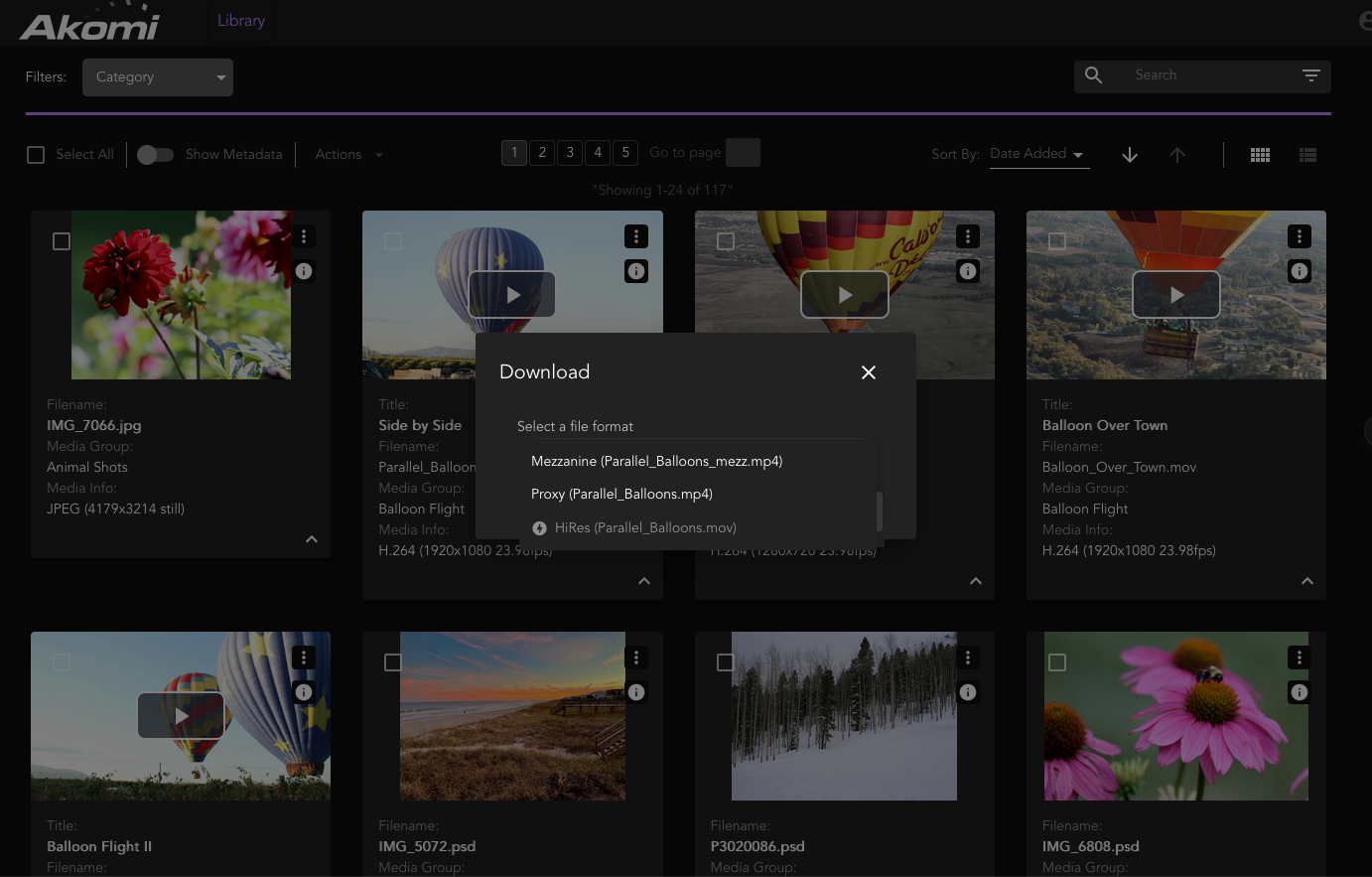The image displays a user interface design set against a black background. In the upper left corner, the text "Okome" is prominently displayed along with a drop-down menu labeled "company." Adjacent to this, there is a magnifying glass icon representing a search function, alongside a search box and a menu icon consisting of three horizontal lines.

A series of navigation elements occupy the top portion, including numbered buttons labeled from 1 to 5, an additional button, and a "sort by" option that comes with its own drop-down menu. Directional arrows (one pointing downwards and another pointing upwards) and a small square icon are also present.

Beneath these elements, there are eight thumbnail images arranged in two rows of four. The top row features images including flowers and three hot air balloons. At the center of these thumbnails lies a black box with the text "Download" and an "X" in the left corner. Inside the box, partially legible text hints at "Select Life Something," although the print is too blurry to read clearly.

The bottom row of thumbnails showcases diverse scenes: one with hot air balloons, a picturesque coastal view with ocean and beaches, a snowy landscape with trees, and a floral display.